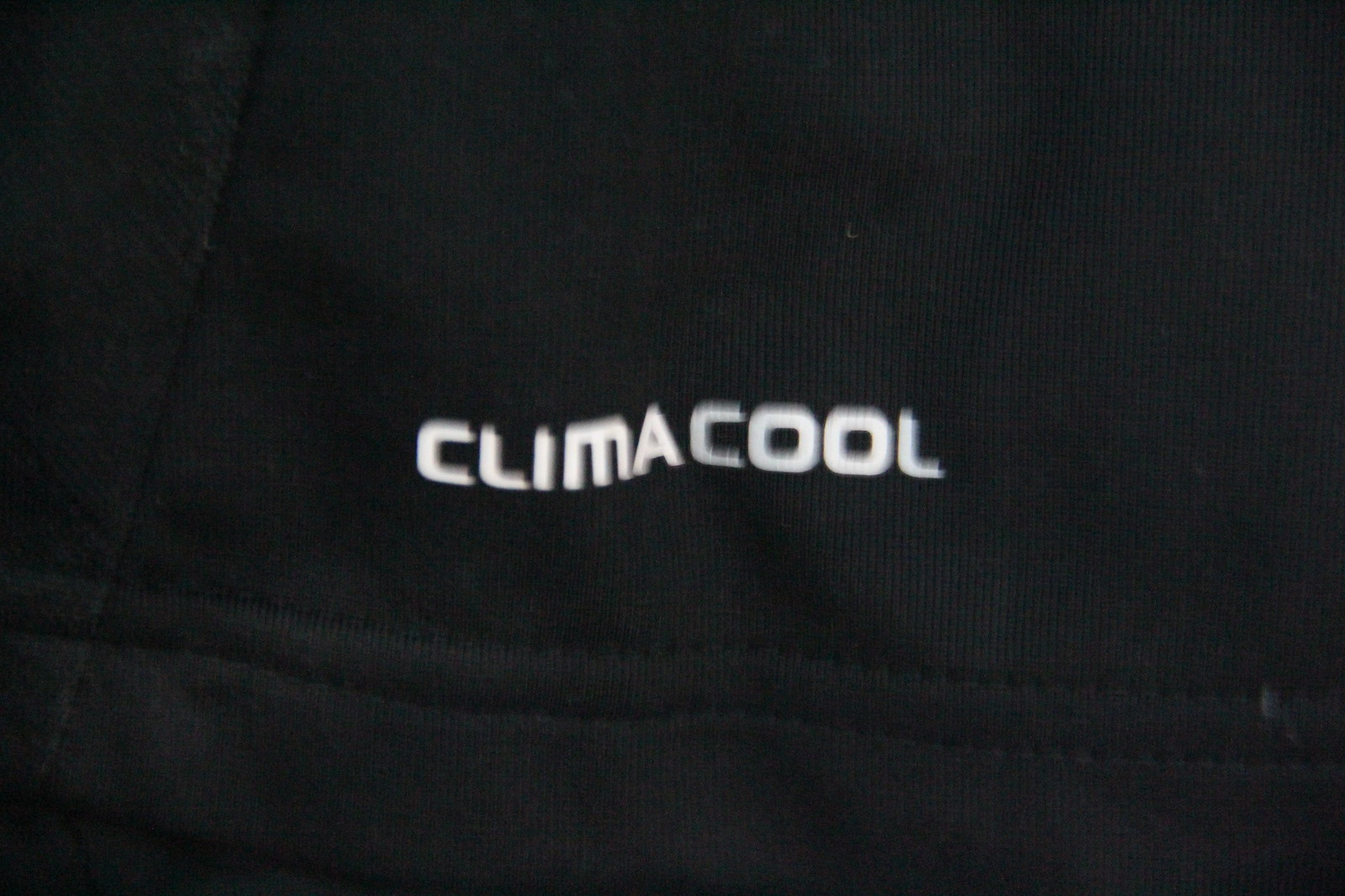This is a close-up image of a black fabric item, completely monochromatic with intricate black stitching. On the left side of the image, a vertical line of thin stitching runs from the top to the bottom, angling slightly toward the bottom left corner. Near the bottom of the image, there is thicker stitching that runs horizontally across the fabric, forming two parallel rows about half an inch apart. There is a small white smudge near the right edge just before the stitching exits the frame. The material shows slight wrinkling but remains predominantly smooth. Centrally positioned is the word "Climacool" in bold white letters outlined in gray, prominently displayed and stitched into the fabric. The overall texture and details of the stitching suggest that this is a carefully constructed textile, possibly a branded piece of clothing.